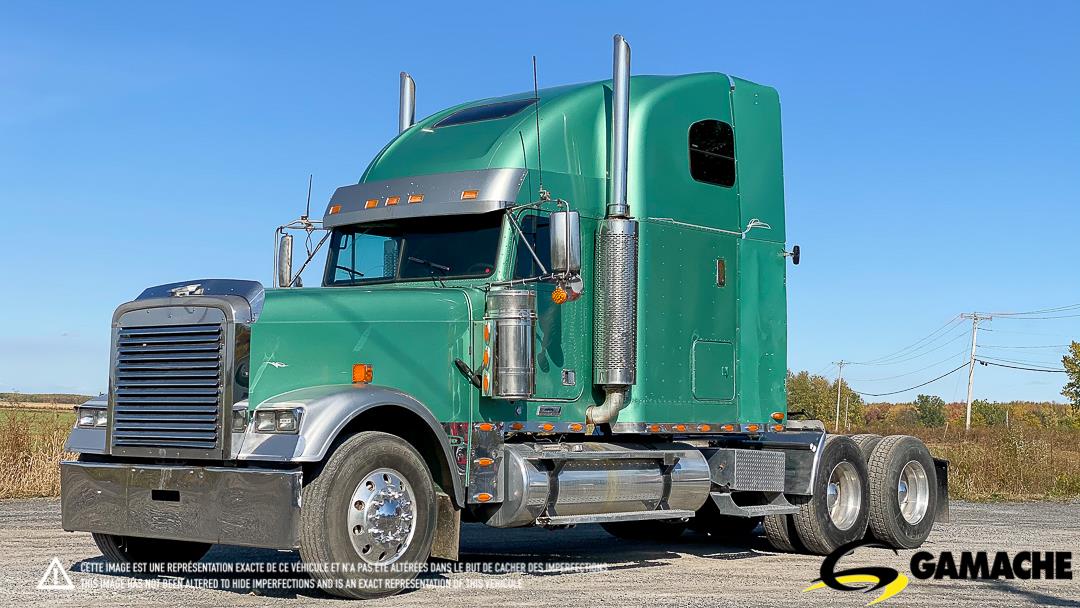In this horizontally aligned rectangular image, the main focus is a large, green semi-truck with shiny teal-green paint and extensive chrome detailing, including a chrome bumper, grill, and fender. The truck features metal-colored silver cylindrical smokestacks on its sides and multiple orange lights scattered around its body. The front end of the semi, positioned towards the left side of the image, is prominently displayed, while the back end extends towards the right.

The truck is parked on a gravel ground with a light and dark gray mixture. In the background, the scene is framed by a large field of grass and trees with no buildings in sight. To the right, there are power lines stretching into the distance. The bright blue sky occupies the entire upper part of the picture, enhancing the image’s vibrant feel.

In the lower right corner, the brand name "GAMACHE" is written in bold, black, all-capital letters. Next to the name, there's a stylized logo featuring a swirled yellow and black design, highlighting the brand identity.